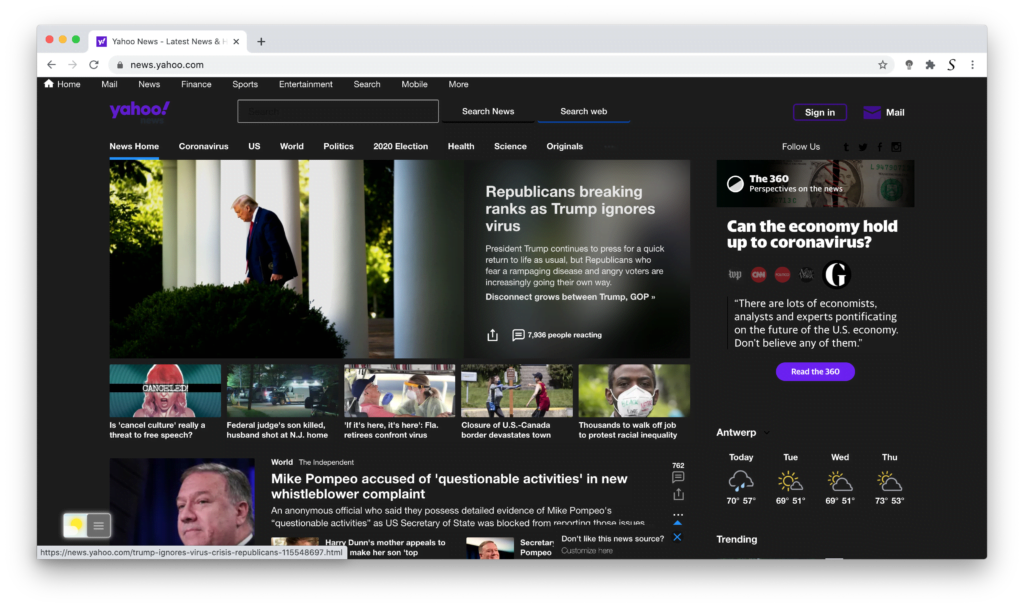The screenshot captures the Yahoo homepage featuring a prominent news story. On the left side of the article, there is an image of Donald Trump walking. To the right of the image, a headline reads "Republicans Breaking Ranks as Trump Ignores Virus." Below the headline, a paragraph states: "President Trump continues to press for a quick return to life as usual, but Republicans who fear a rampaging disease and angry voters are increasingly going their own way." Adjacent to this article, there is another headline questioning, "Can the Economy Hold Up to Coronavirus?" This section mentions the opinions of various economists, analysts, and experts about the future of the U.S. economy, followed by the advice to be skeptical of their predictions. A prominent blue button is located below this text.